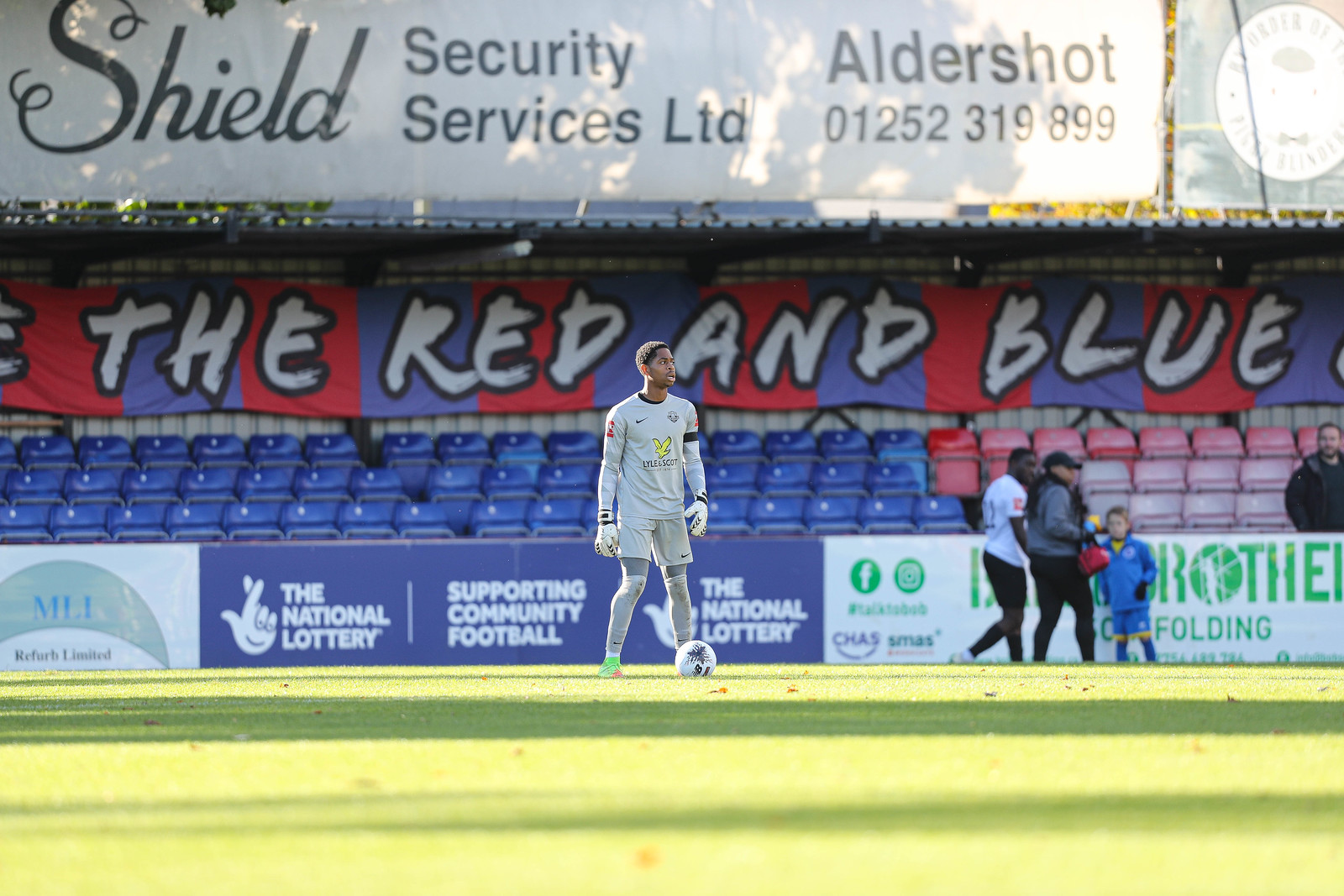This color photograph captures a young boy standing alone on a soccer field, dressed in a pristine white athletic uniform. Positioned at his left foot is a white soccer ball. His gaze is directed off towards the distance to his left, creating a contemplative mood. The stadium surrounding him is completely empty, revealing rows of alternating red and blue seats. In the background, three distant figures walk along the perimeter of the field. Above the seats, a banner prominently displays the text "The Red and Blue," alongside several advertisements, including “Shield Security Services Limited, Aldershot 01252 319 899” and “The National Lottery, Supporting Community Football.” The photograph is taken outdoors during daytime, highlighting the vibrant colors of red, white, blue, and various shades of green from the grass field. Additional advertisements can be seen on the top edges of the stadium, tying into the overall theme of community and sportsmanship.